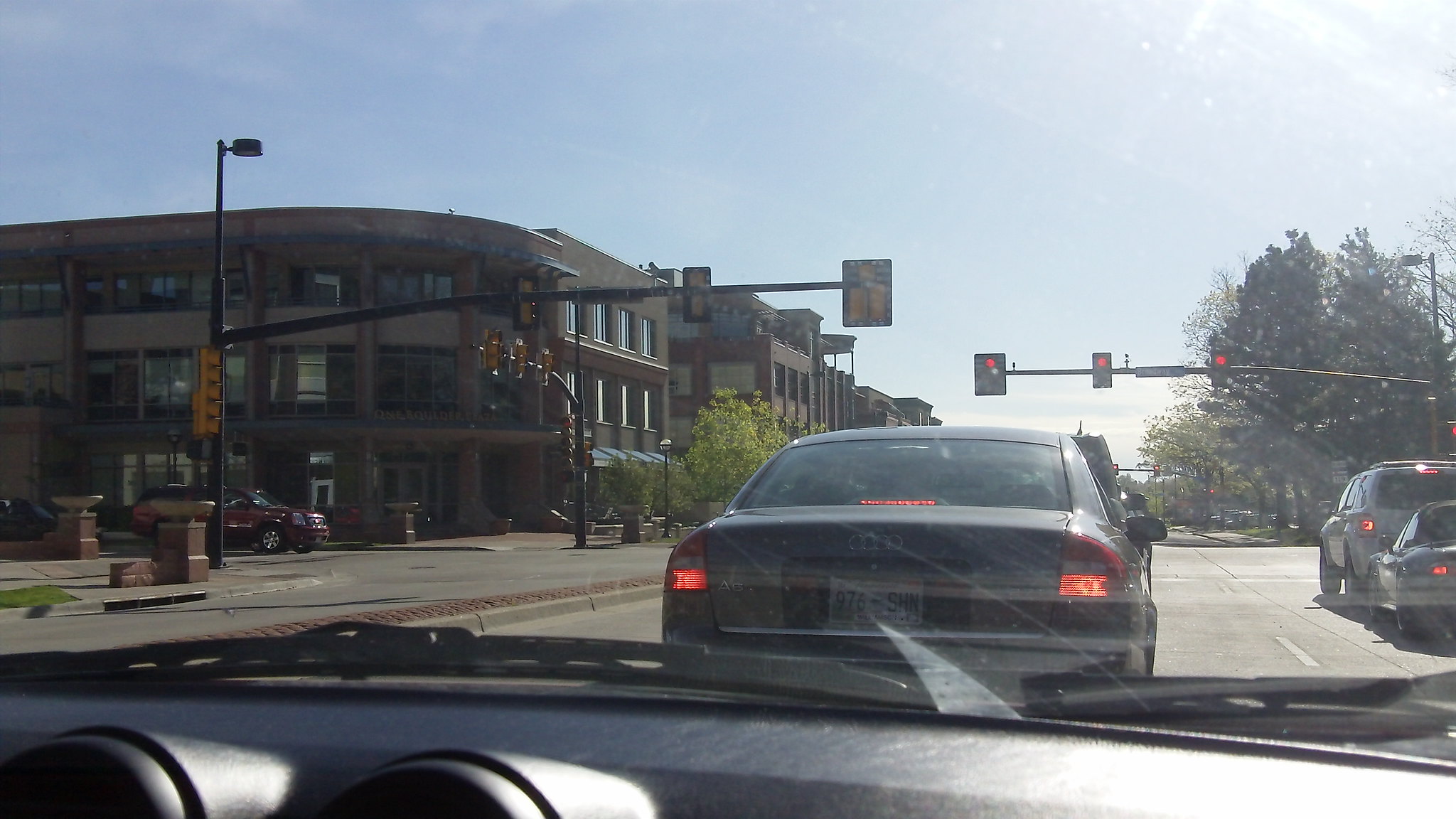The photo captures a vivid scene of two cars awaiting a green light at an intersection on a bright, sunny day. Snapped from the interior of another vehicle, potentially from the driver’s perspective, the image offers a detailed peek into the car's shadowy outline and reflections. The wide road, indicative of North American landscapes such as Canada or the United States, hosts large SUVs parked at the roadside. In the backdrop, a grand brown building with large windows and transparent door panels adds character to the urban setting. Flourishing green trees and a water fountain contribute to the scene's lively atmosphere, making the whole composition dynamic and visually engaging.